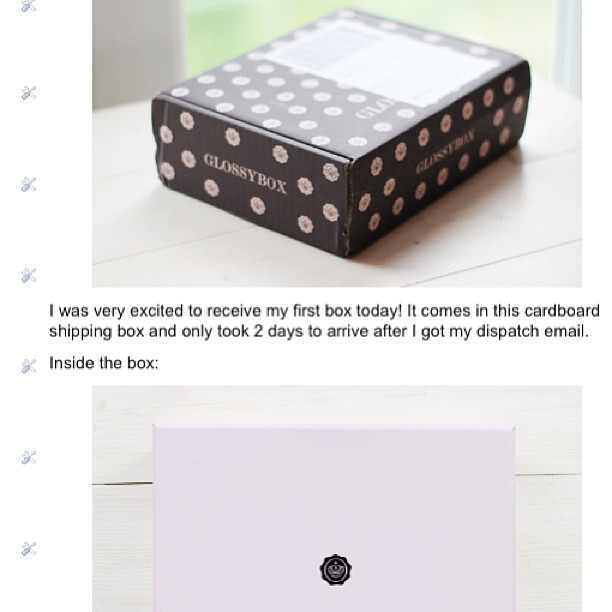This detailed caption summarizes the description of the image:

"This image is a tall rectangular screenshot of a review on a website, featuring a predominantly white background. On the top left corner, a vertical pattern of tiny cartoons of a crossed screwdriver and wrench descends evenly down the page. The main content is divided into two sections with a block of black text in the center. The top section displays a diagonally oriented photograph of a brown Glossybox with light pink flowers, positioned on a white wooden surface. The box is shown with one side facing the lower left corner and the other side facing the top right corner of the image. The black capital letters 'GLOSSYBOX' are visible on the side of the box. Beneath this image, the text reads: 'I was very excited to receive my first box today. It comes in this cardboard shipping box and only took two days to arrive after I got my dispatch email.' The bottom section shows another image, this time of an envelope on the same white wooden surface. The envelope appears to be slightly pink and features a seal that possibly displays the company logo."